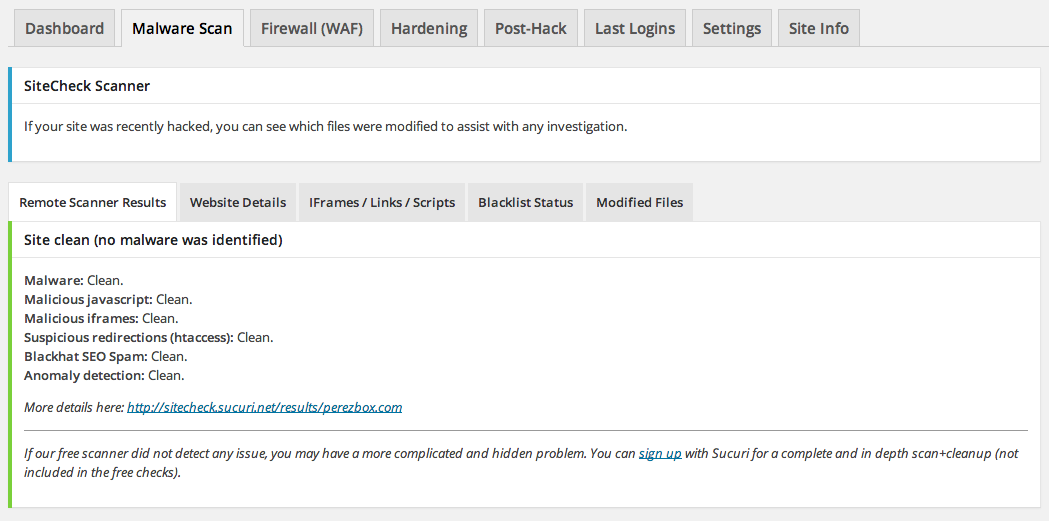### Detailed Descriptive Caption

This image features a computer program interface open to the 'Malware Scan' tab. At the top of the window, a series of navigation tabs are visible, labeled from left to right as follows: Dashboard, Malware Scan, Firewall, Hardening, Post Hack, Last Logins, Settings, Site Info. The currently selected tab is 'Malware Scan'. 

Beneath it, there is a section labeled 'Site Check Scanner', which offers functionality for reviewing modified files if a site was recently hacked to assist with investigations. Below this section is another panel with a set of tabs. These tabs are: Remote Scanner Results, Website Details, iFrames/Links/Scripts, Blacklist Status, and Modified Files.

The active tab in this section is 'Remote Scanner Results'. Within this tab, there is a message indicating the site is clean – "Site Clean, no malware was identified." Following this, a comprehensive list of statuses is shown:
- **Malware:** Clean
- **Malicious JavaScript:** Clean
- **Malicious iFrames:** Clean
- **Suspicious Redirections:** None
- **HT Access:** Clean
- **Black Hat SEO Spam:** Clean
- **Anonymous Detection:** Clean

At the bottom of this list, there is an option to view more details, highlighted by text that says "More Details here", which is presented as a clickable blue hyperlink directing to a website.